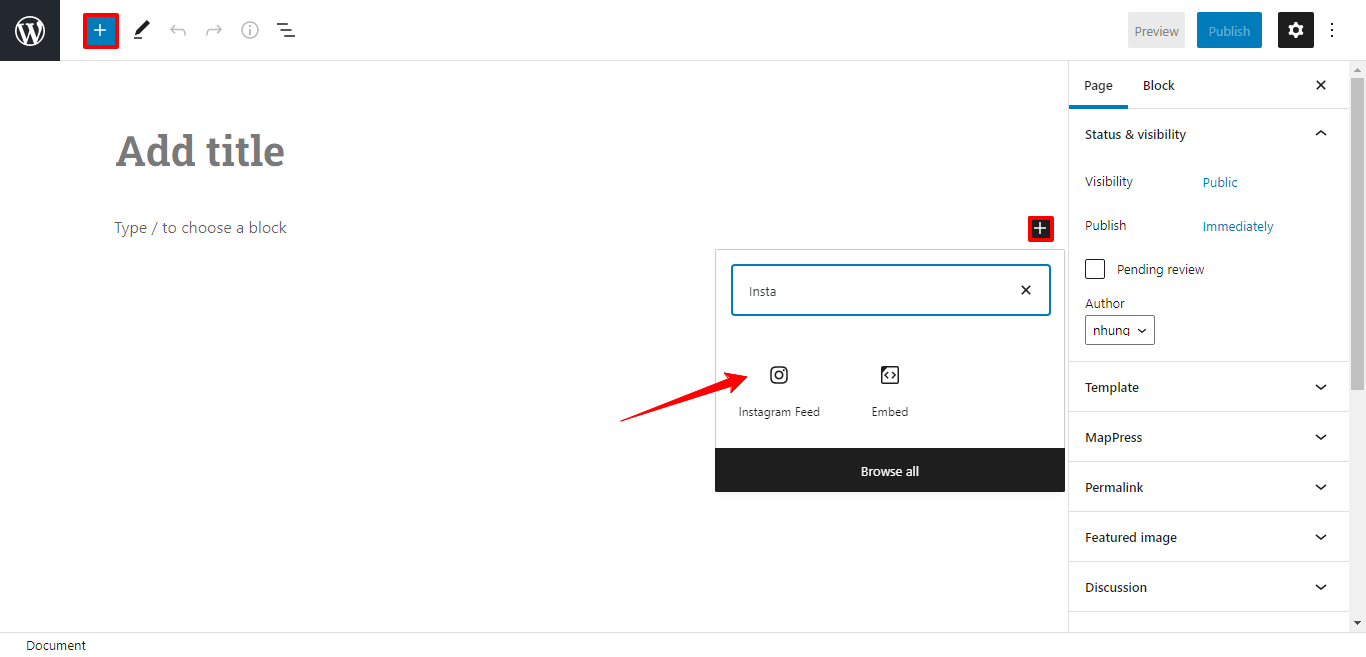This image is a detailed screenshot of the admin section of a WordPress website, specifically the content creation page. Featured prominently in the top left corner is the WordPress logo: a black square with a white "W" encircled. This iconic logo represents WordPress, a leading website builder used by over 20% of the world's websites.

The background of the page is a clean, minimalist white, providing a clutter-free workspace. At the upper left, the page title section prompts users with the text "Add title," indicating where the article or blog post's title should be placed. Below this, there is space allocated for writing the main content.

On the right side of the screen, a sidebar offers several functional options. This includes dropdown menus for selecting a template, configuring MapPress settings, setting the permalink, assigning a featured image, and managing discussion settings. Adjacent to this sidebar is a grayed-out outlined square, which appears to serve a specific function within the admin interface. At the bottom of this square, a black button stretches horizontally, labeled "Browse all" in white text, inviting users to explore additional options or media.

This screenshot effectively captures the intuitive design and user-friendly interface that WordPress provides for content creators.